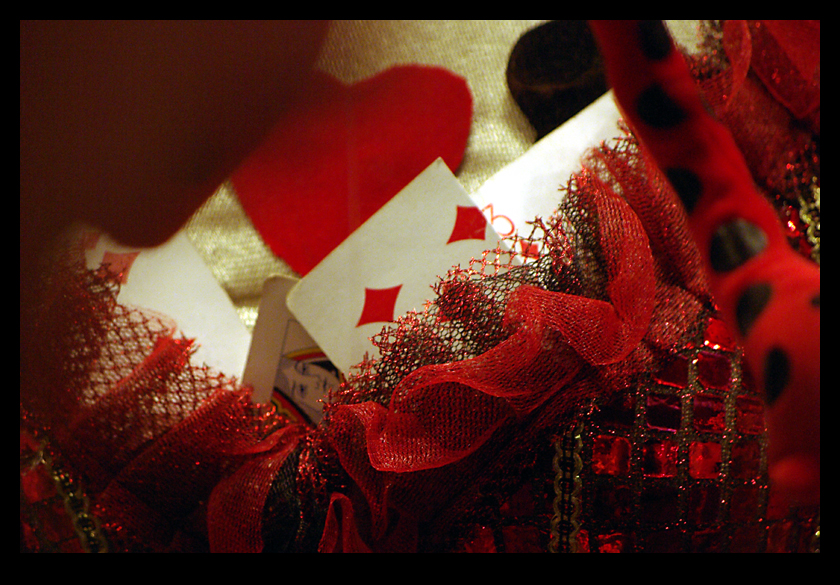This vibrant color photograph captures a visually rich scene set on a cozy brown blanket. Scattered across the blanket are four playing cards: a three of diamonds, a queen, and two partially visible cards. Among these cards lies a plush, red heart-shaped fabric piece. The heart, adorned with glitter, adds a touch of whimsy to the image.

A dazzling, sequined hair bow occupies the center of the picture, emitting a shiny, reflective quality that dominates the composition. To the right of this glittering accessory, a pair of equally sparkly red gloves enhance the overall festive atmosphere.

In the upper left-hand corner, the shadow of a person partially obscures the details of one playing card, adding an element of mystery. Nestled beside the fabric heart, towards the center of the frame, is a small, round purple object that resembles a ball of fabric, contributing to the texture-rich tableau.